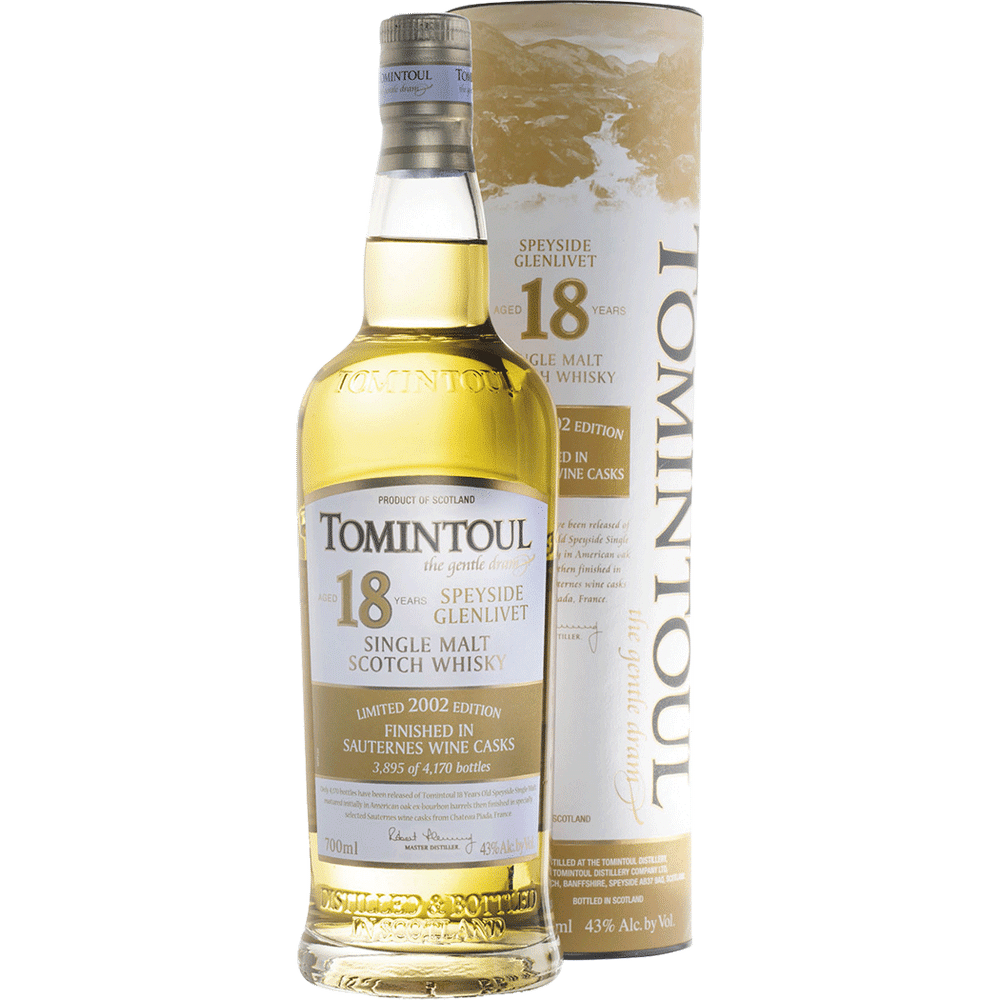The image depicts a bottle of Tomintoul 18-Year-Old Single Malt Scotch Whisky standing in front of its cylindrical cardboard container. The whisky itself is a pale, light golden hue, corresponding to the elegant white label adorned with beige and dark grey text. It proudly announces its 18 years of aging and its unique finish in Sauternes wine casks. Notably, this limited 2002 edition bottle is marked as number 3,895 out of a total of 4,170, emphasizing its exclusivity. The label also highlights the whisky's origin as a product of Scotland and its 43% alcohol by volume content. The packaging and presentation make it an ideal and likely expensive gift, with the cylindrical container adding a distinctive touch compared to the more common box or bag. The background of the image is white, partially cutting off the top, and the bottle appears unopened and full, suggesting it is in pristine condition.